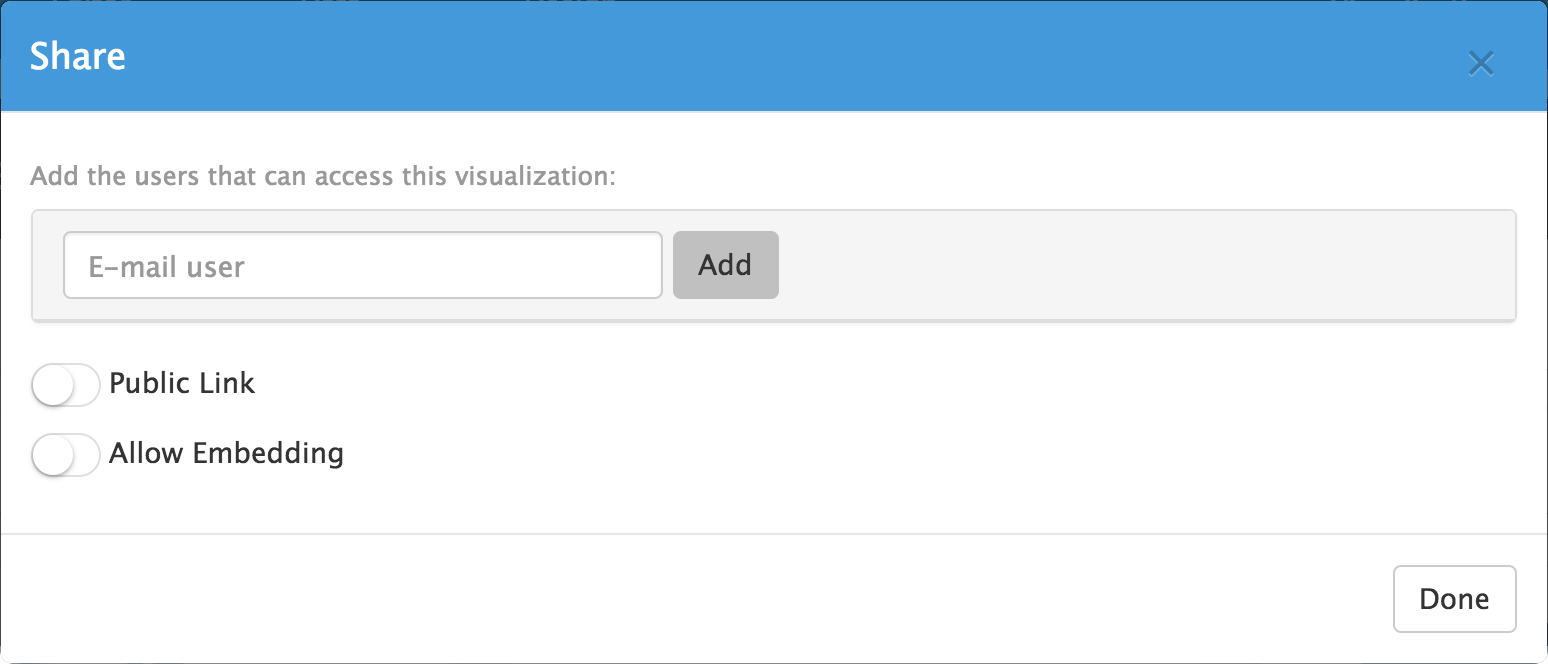The image depicts a computer interface window predominantly featuring a stark white background. At the top of this window is a distinctive blue bar, labeled "Share" in white letters situated in the left corner. The right corner of this blue bar contains a standard "X" button for closing the window.

Below the blue bar is a prominent white box that serves as the main content area. At the top of this white box, there is an instructional text in black that reads, "Add users that can access this visualization." Directly beneath this text lies another smaller, light gray box which houses an input field. This input field is also white and contains placeholder text that says "Email user."

Adjacent to this email input field, there is a smaller, gray box featuring the word "Add" in black lettering, indicating a button function to add the email user specified.

Further down the interface, there is a slider bar accompanied by options labeled "Public link" and "Allow embedding," suggesting adjustable sharing settings.

At the very bottom of the window, a thin blue line separates the content from the footer. Positioned in the right corner of this footer area is a button labeled "Done."

Overall, the interface is minimalistic and uses a limited color palette consisting of blue, gray, white, and black. The design is straightforward and devoid of any extraneous elements beyond the described features.